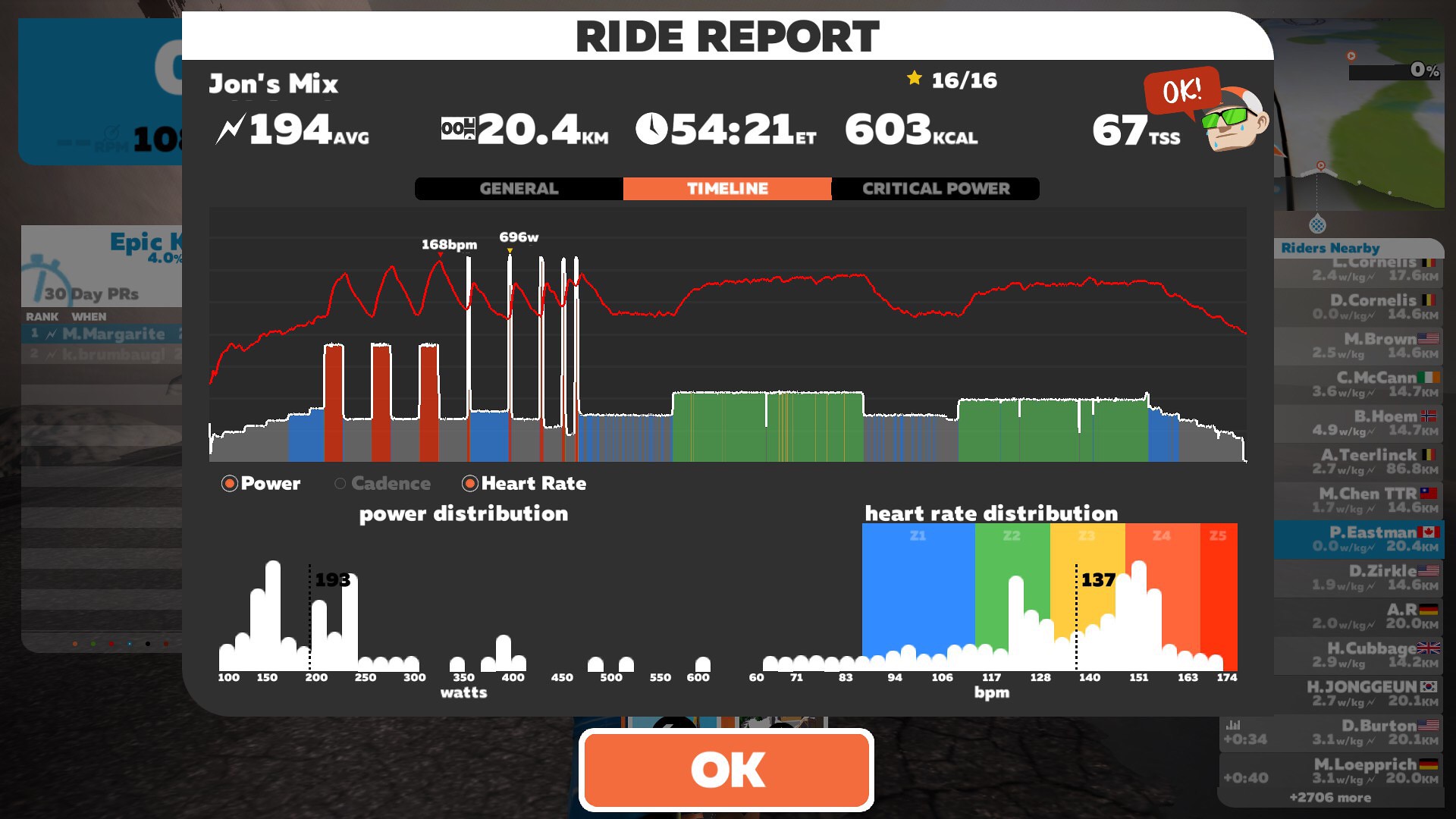The image depicts a detailed "Ride Report" graph with multiple types of data visualization. At the top of the report, the header reads "Ride Report" in black text on a white background. On the left side, it’s labeled "John's Mix," indicating the specific ride or workout. Directly to the right, several key statistics are prominently displayed: an average of 194, a distance of 20.4 KM, an elapsed time (ET) of 54:21, a caloric expenditure of 603 Kcal, and a Training Stress Score (TSS) of 67.

The upper right-hand corner features a cartoon man's face wearing a red and white hat with green glasses, accompanied by a red conversation bubble with the word "OK" inside. Below this image, there are buttons titled "general timeline" and "critical power," which allow viewers to switch between different versions of the graph.

The main graph/chart area showcases a red line graph alongside bar graphs composed of red, blue, green, and gray bars. Categories such as power, cadence, heart rate, power distribution, and heart rate distribution are indicated, each with corresponding graphical bars. Below these categories, there is another "OK" button.

Additionally, a list of names, likely representing nearby riders or participants, is visible on a gray and blue background on the right side of the image. The names include Pete Eastman (Canada), L. Cornett, D. Cornelius, M. Brown, C. McCain, B. Holm, A. Tierlink, M. Chen, D. Zirkle, H. Cubbings, H. Jonaghan, D. Burton, and M. Ludin-something.

Overall, this report provides a comprehensive snapshot of John's ride, offering various performance metrics and visual summaries through line and bar graphs, all set against a dark gray backdrop for easy readability.